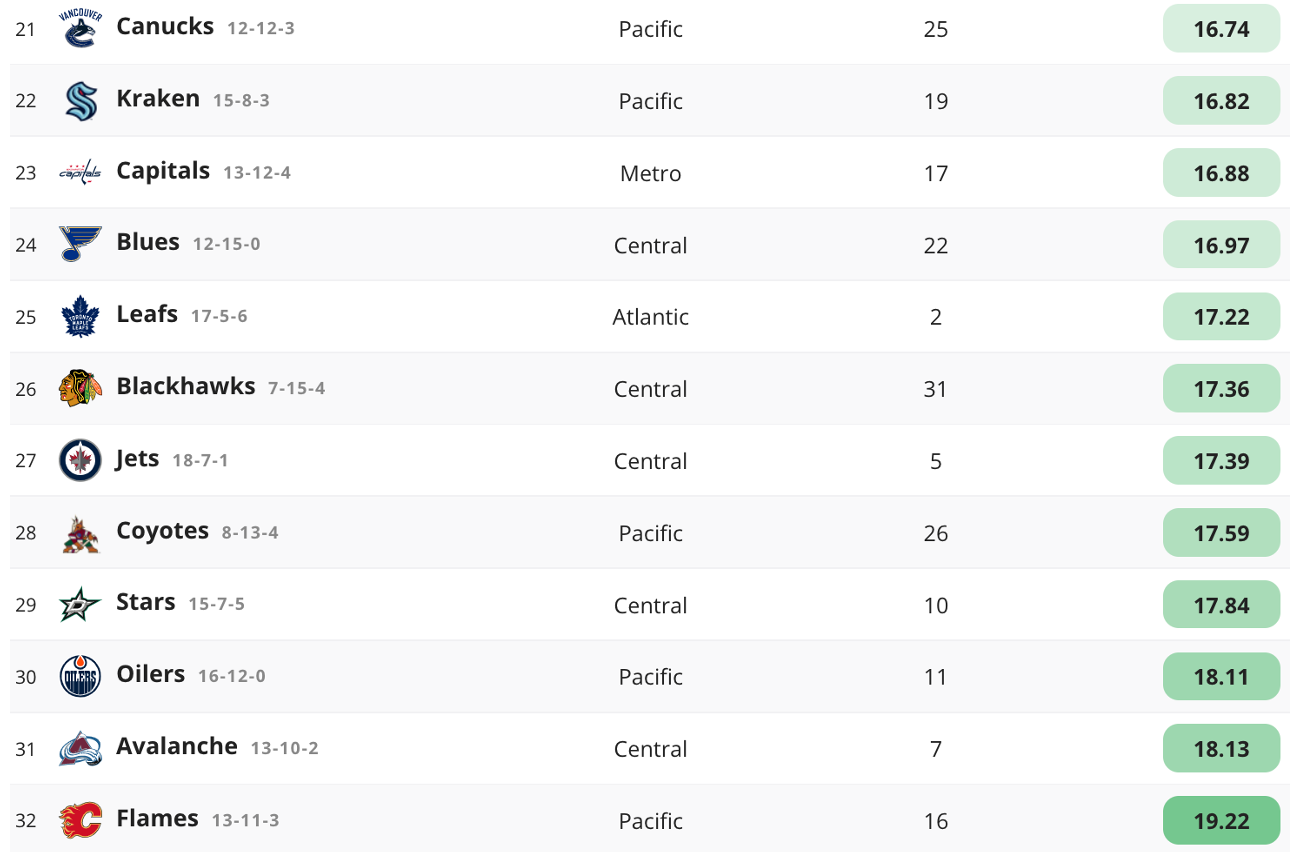This screenshot, from an unspecified source, showcases a detailed list of several sports teams along with their standings and statistics. The information is organized by team name, their win-loss-overtime records, division, rank, and some form of rating or score:

1. **Canucks**: Record: 12-12-3, Division: Pacific, Rank: 21, Score: 16.74
2. **Kraken**: Record: 15-8-3, Division: Pacific, Rank: 19, Score: 16.82
3. **Capitals**: Record: 13-12-4, Division: Metro, Rank: 17, Score: 16.88
4. **Blues**: Record: 12-15-0, Division: Central, Rank: 22, Score: 16.97
5. **Leafs**: Record: 17-5-6, Division: Atlantic, Rank: 2, Score: 17.22
6. **Blackhawks**: Record: 7-15-4, Division: Central, Rank: 31, Score: 17.36
7. **Jets**: Record: 18-7-1, Division: Central, Rank: 5, Score: 17.39
8. **Coyotes**: Record: 8-13-4, Division: Pacific, Rank: 26, Score: 17.59
9. **Stars**: Record: 15-7-5, Division: Central, Rank: 10, Score: 17.84
10. **Oilers**: Record: 16-12-0, Division: Pacific, Rank: 11, Score: 18.11
11. **Avalanche**: Record: 13-10-2, Division: Central, Rank: 7, Score: 18.13
12. **Flames**: Record: 13-11-3, Division: Pacific, Rank: 16, Score: 19.22

This organized format highlights each team's performance metrics comprehensively, providing a clear view of their standings within their respective divisions.